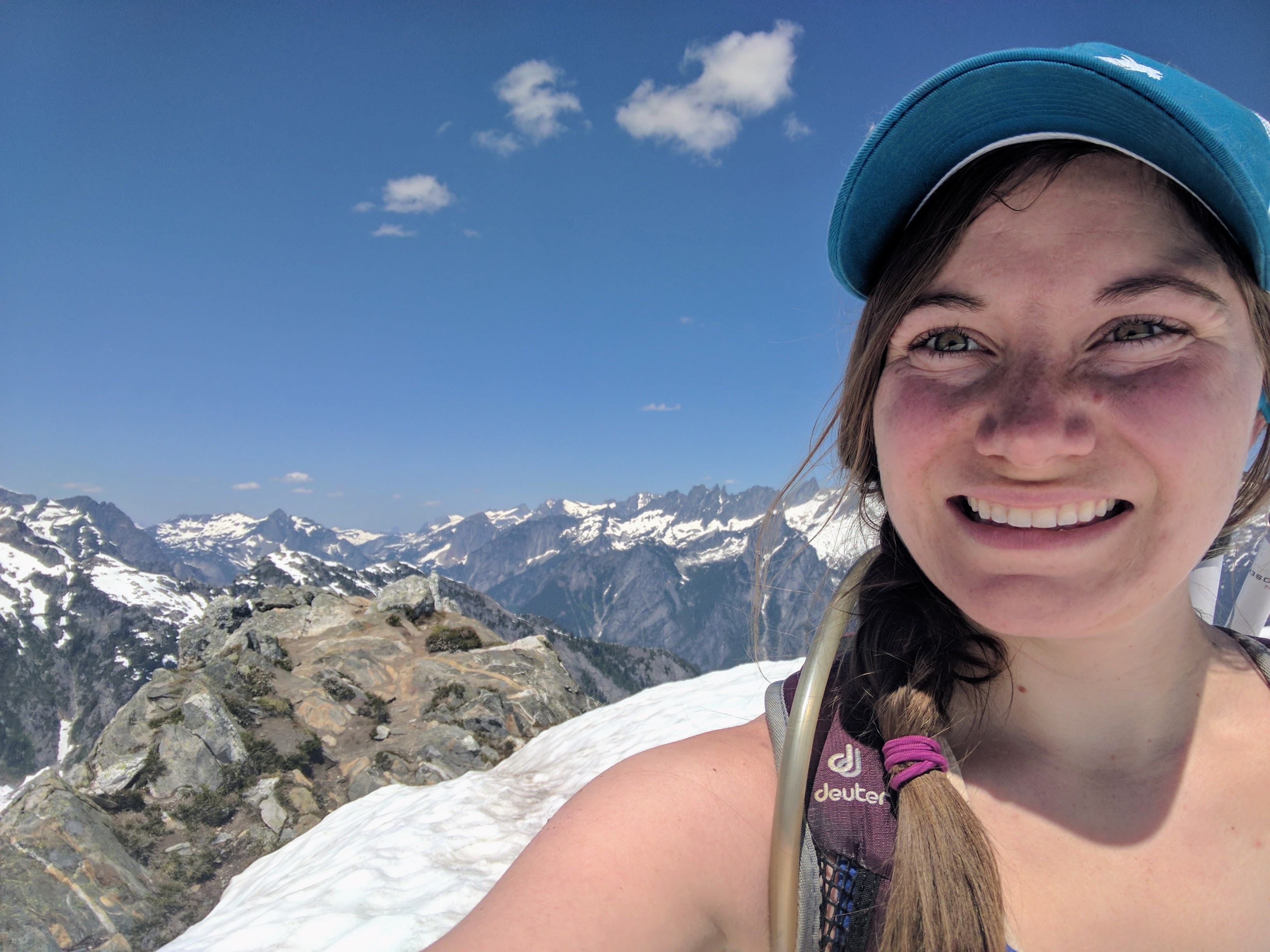This vibrant square selfie captures a cheerful woman positioned on the right side. She's wearing a light blue ball cap, her straight brown hair pulled back over her shoulder in a ponytail secured with a purple band. Her broad smile reveals her teeth, and although she isn’t quite looking at the camera, her joy is palpable. She sports a backpack, with the visible strap on her shoulder subtly marked with the word "Deuter." Her attire includes a low-cut blouse, hinting just at her neckline and shoulder, adding a touch of casual style. Behind her stretches a stunning expanse of nature: a clear blue sky with a few feathery white clouds above a majestic mountain range. The closer mountains display varying shades of gray and brown, some peaks capped with pristine white snow, emphasizing the grandeur of her high-altitude location. This mosaic of elements enhances the portrait with both personal charm and the awe of the surrounding natural beauty.